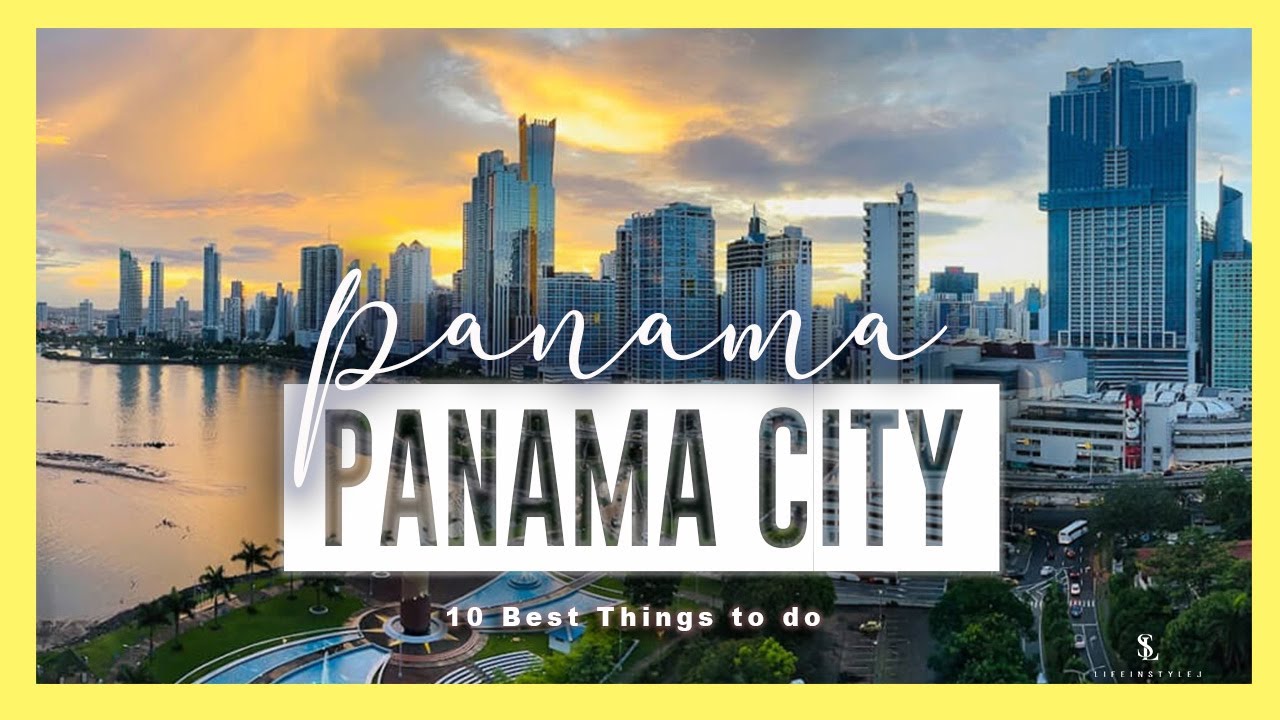The image captures a vibrant cityscape bathed in the warm hues of a setting sun, with clouds scattered, especially in the top left corner. The scene is bordered by a neon, yet very light yellow outline. On the right side of the image stands a prominent rectangular building with a flat facade. The exterior is light silver, but the face appears as a dark chrome. In the middle center of the image, white cursive lettering spells out "Panama" with considerable spacing between the connected letters. Below this, a label-style banner with a white background features capital block letters that are transparent, allowing the background image to show through. The text reads "PANAMA CITY" and underneath it in white lettering, it states "10 best things to do," also with noticeable spacing.

Towards the bottom right, a white logo resembling a Times New Roman font similar to the Yves Saint Laurent logo is present. It consists of a white 'S' with an uppercase 'L' intersecting through it. Below this, it reads "LIFE IN STYLE J" in uppercase white letters, again with distinctive character spacing. To the left of this logo (still at the bottom right of the image), a road is visible, populated with several vehicles including a notable white bus towards the right. In the background of the road, either a large white building or a ship is discernible.